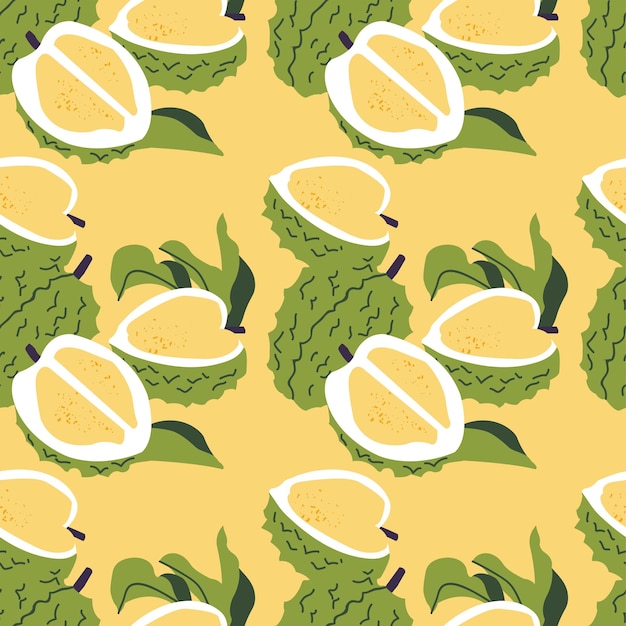The image depicts a repeating pattern of a stylized tropical fruit, likely meant to represent a guava or durian, though it's not a clear depiction of any specific real fruit. The background is a pale yellow that matches the yellow flesh of the fruit displayed. The fruit, depicted both whole and cut open, has a green, textured, and spiky exterior with small green leaves sprouting from the top. When cut open, the interior reveals a soft, yellow flesh with a distinct white line running through the center, resembling deviled eggs in coloration. All in all, the image consists of a beige, white, yellow, and green color palette, forming an endless, repeating pattern that appears similar to wallpaper or wrapping paper.